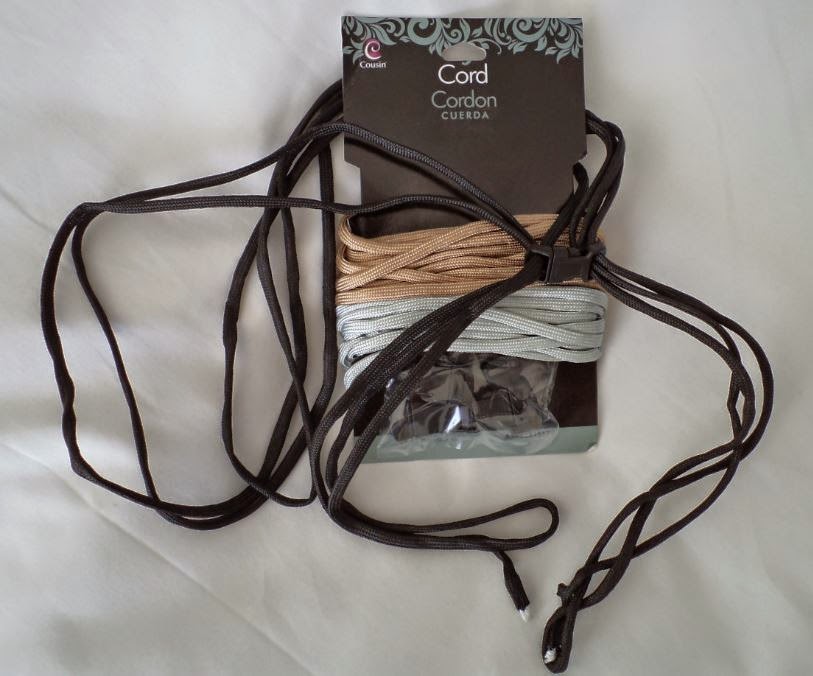The image is a detailed, staged photograph taken indoors, featuring a package of fabric cords displayed against a light gray, wrinkled cloth backdrop. The package itself is a brown rectangular piece of cardboard adorned with gray, leaf-like swirly designs at the top. Prominently displayed on the package, the word "cord" appears in white, while "cordon" and "cuerda" are printed in silver, indicating three different languages. The package, branded with the "Cousin" logo, contains a variety of cords: a neatly wrapped light brown cord, a neatly wrapped light gray cord, and a dark brown cord that is somewhat haphazardly wound and extends around the item. The package also features clear tape at the bottom, suggesting it was used to secure the cords in place.